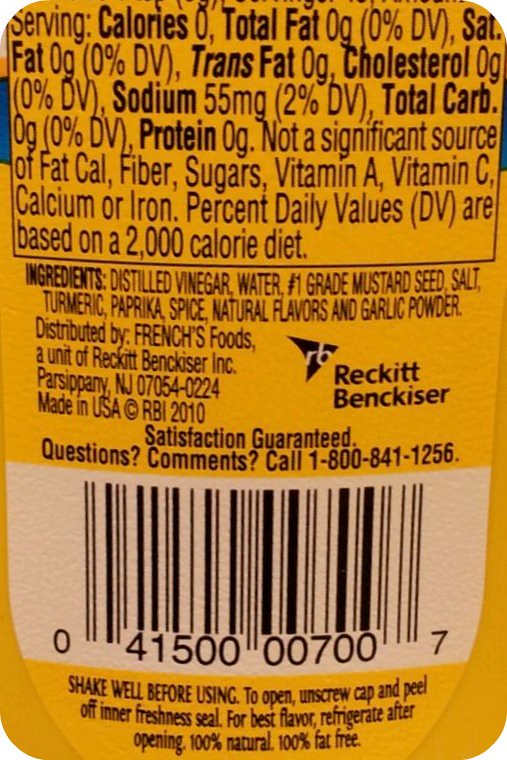Here is a detailed and cleaned-up caption:

---

This image displays the backside label of a product from Reckitt Minsker, featuring detailed ingredient information. The label's color is a rich pumpkin orange. Positioned at the bottom is a white barcode with the number 4150000700. The ingredients, written in capitalized black text, include distilled vinegar, water, mustard seed, salt, turmeric, paprika, and additional spices. The nutritional information indicates that the product contains zero calories, zero fat, zero trans fat, and 55 milligrams of sodium. The label advises users to "shake well before using." Distributed by French's Food, this appears to be a bottle of Worcestershire sauce based on the ingredients listed.

---